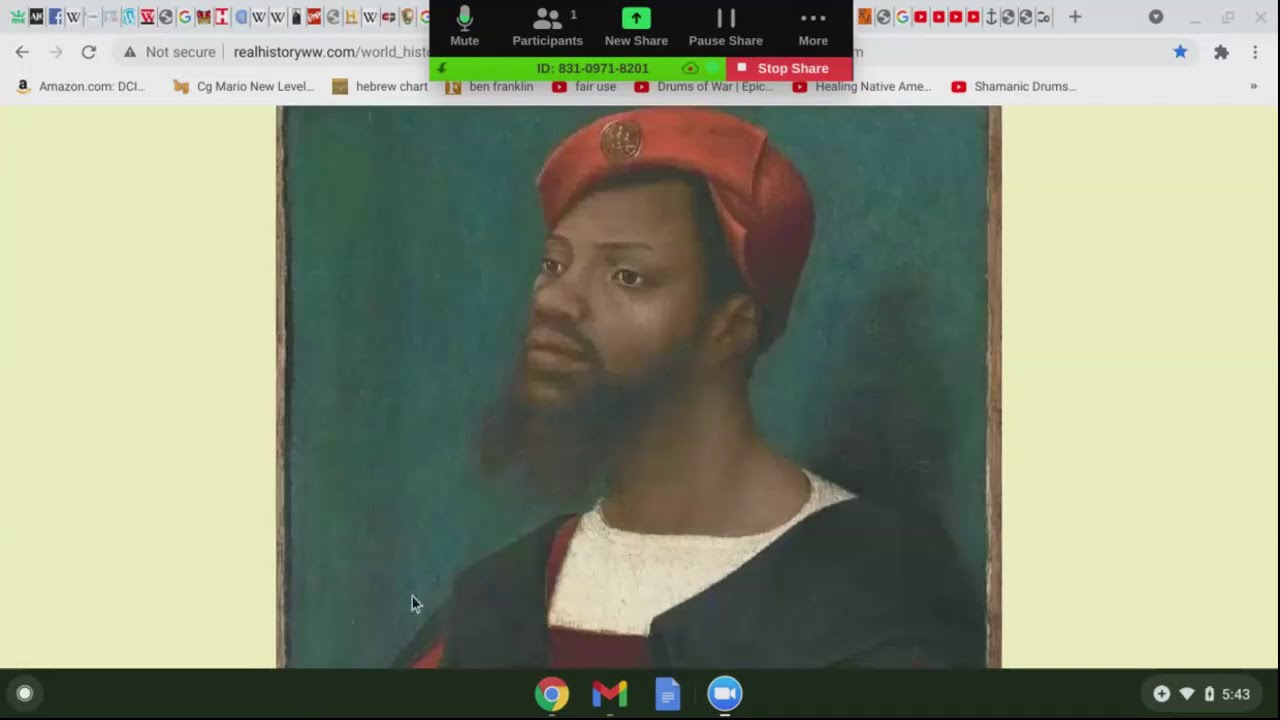The screenshot captures a computer screen with a focused view on a detailed painting displayed on a website. The computer appears to be a Mac, and the screenshot is taken from a web browser, specifically on the site realhistoryww.com, indicated to be an unsecured site, as shown by the "not secure" icon in the top left corner. The top border of the image features a browser bar with numerous bookmarked icons and a player overlay that includes options such as 'mute participants,' 'new share,' 'pause share,' and more, indicative of a video call being in progress. The bottom border has a black rectangular strip with various application icons like Google Chrome, Gmail, Google Voice, and a video clip icon. The clock in the right-hand corner shows the time as 5:43, along with the battery life, confirming it's a laptop. 

At the center of the screen is a striking painting against a yellow backdrop. The painting depicts a black man with a bushy black beard, wearing a distinctive red round hat adorned with a gold seal on top. He is dressed in a black robe draped over a white shirt with a burgundy trim and is set against a green background. The man in the painting is looking off to the side, presenting a profile view suggestive of historical portraiture, possibly from the 16th or 17th century.